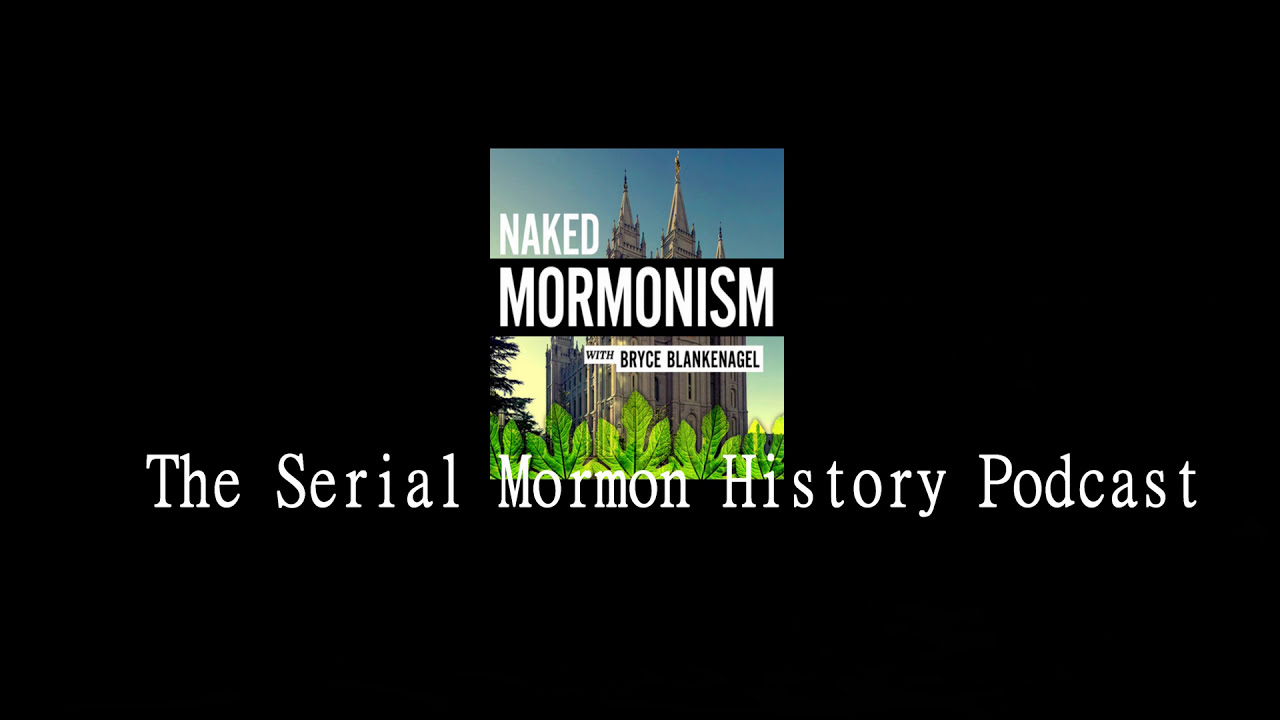The image is a black rectangle, likely an advertisement for a podcast titled "Naked Mormonism." In the center, there is a square image of an ornate, cathedral-like building with a realistic appearance, set against a blue sky. Prominently in front of the building are large green leaves, which appear to be drawn. The title "NAKED" is in bold white uppercase sans-serif text, positioned above the word "Mormonism," which is also in white but set against a black rectangle. Beneath the title, in a white text box, is the name of the podcast host, "With Bryce Blankenagel." Below the square image, in a serif font, the description reads "The Serial Mormon History Podcast," in white letters, each word capitalized. The entire composition sits within a thick black border, giving it the appearance of a polished, intentional design, possibly a thumbnail for the podcast.